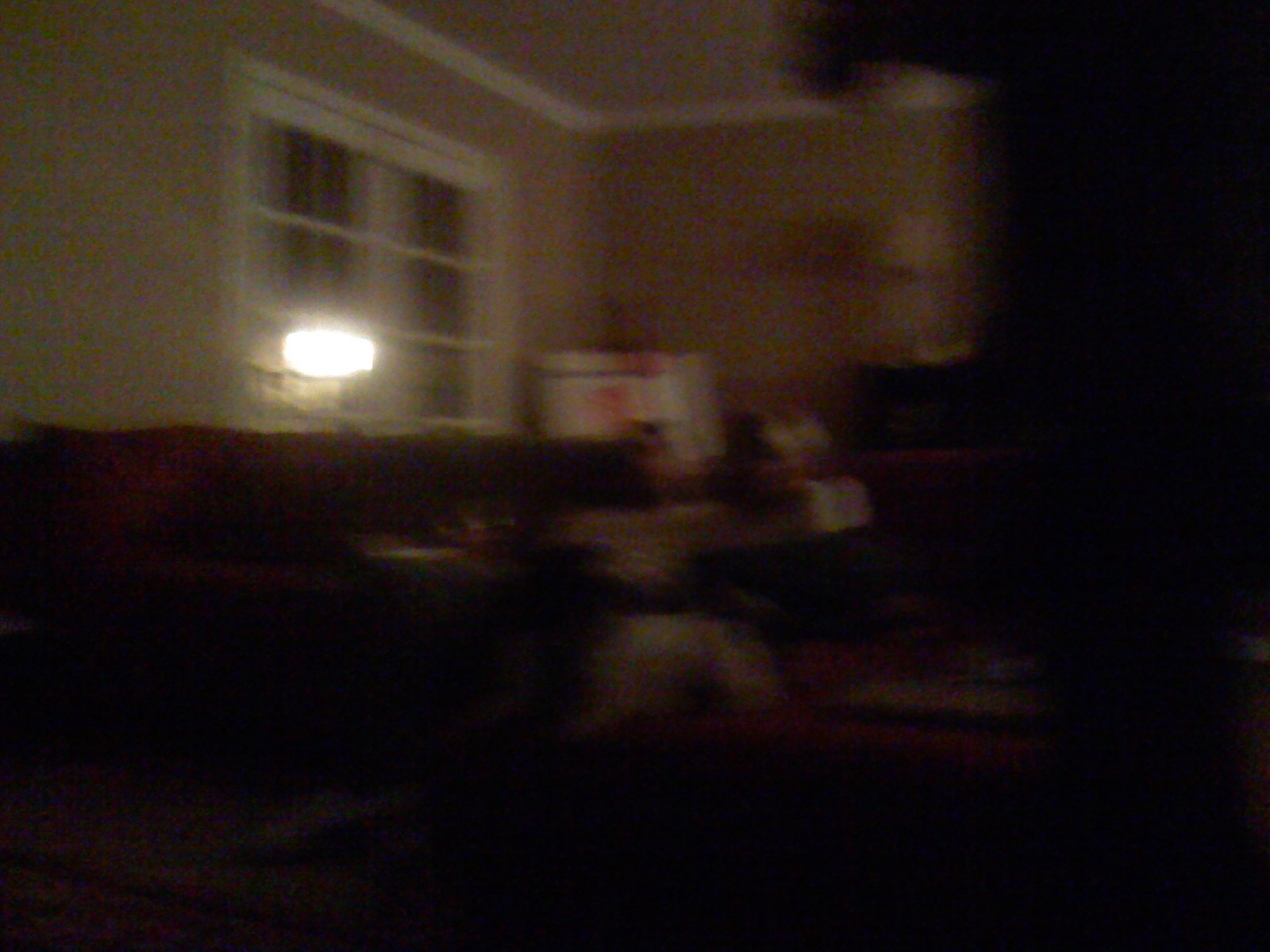This is a blurry color photograph taken inside a living room of someone's home at night. The image features a large white triple-pane window with a small lamp on in front of it, casting an oval light into the room. The walls appear to be a greenish-tan color with white trim around the corners of the ceiling. A burgundy or dark red L-shaped couch is visible, with a red blanket draped over the back on the left-hand side. The flooring is a brownish-beige carpet. There appears to be an area rug of a similar reddish hue beneath the couch. In the image, you can see a white box with some red on it in the corner of the room and papers strewn about on a table or the couch. There is some indication of people in the room, with one person seemingly sitting in a chair wearing a dress, and another possibly sitting on the carpet. The scene appears cluttered with various whitish objects scattered throughout the room. The photograph is dark and very blurry, making it difficult to discern finer details or additional elements in the space.